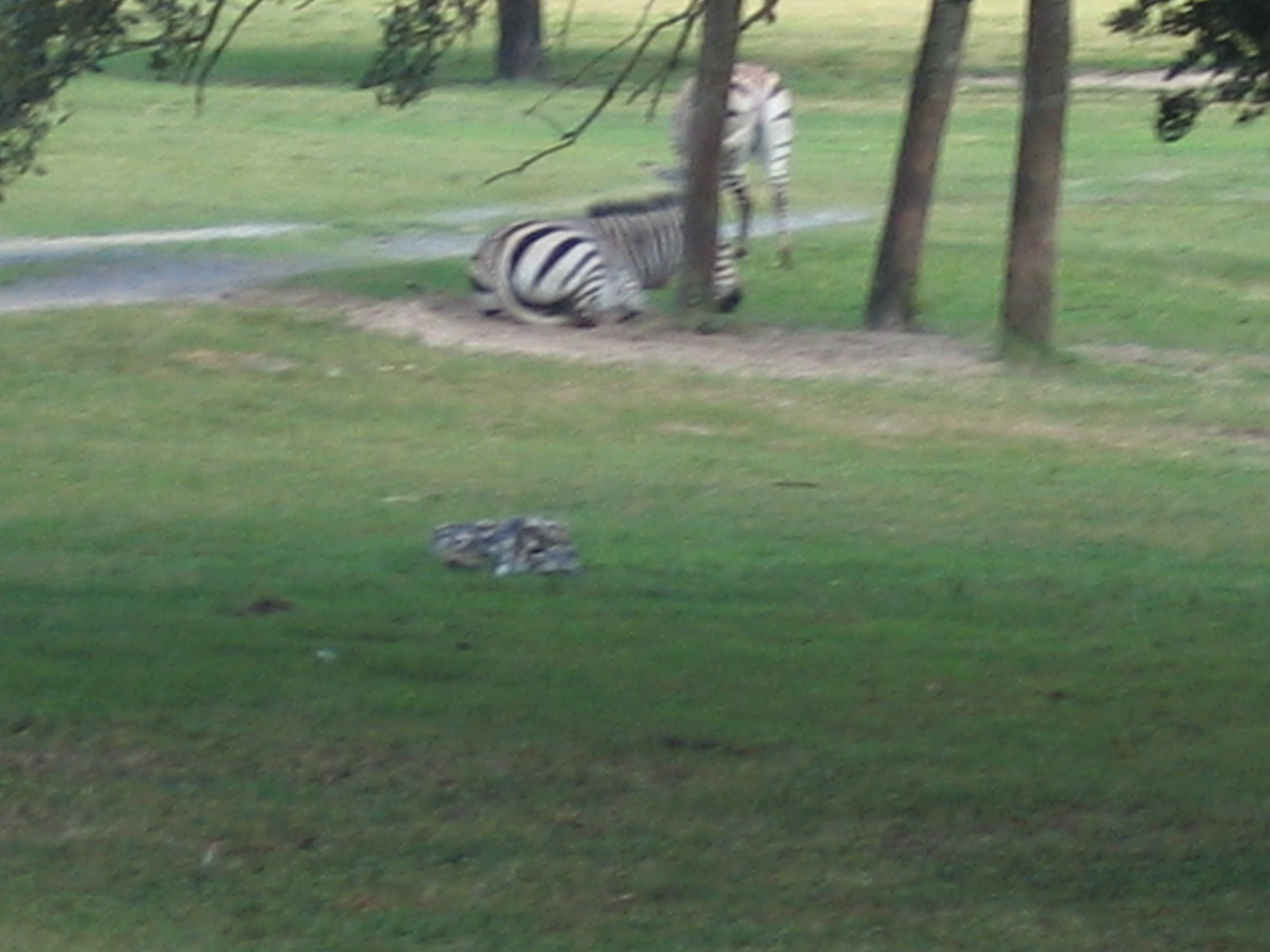This is a slightly blurry photograph taken outdoors, featuring two zebras in a grassy area with some patches of brown. Neither zebra is in the foreground; both are positioned towards the middle background of the image. One zebra is standing with only its rear visible, and the other zebra is lying on its side, providing a good view of its profile and part of its face, including its short black mane and distinctive black and white stripes. A slender tree trunk stands in front of the zebras, partially obscuring them. Scattered throughout the image are additional tree trunks and branches, none fully visible. The foreground consists mainly of grass, with some worn-down paths, possibly created by frequent zebra activity. There's also a barely distinguishable, out-of-focus gray object on the ground, which could be a rock.